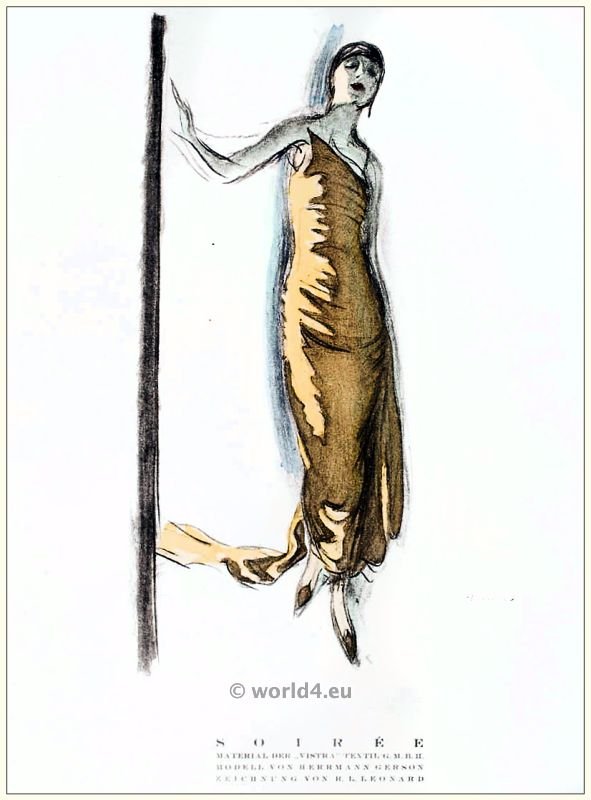The image depicts a stylish, high-fashion poster featuring a slender, white model with pale skin, dressed in an asymmetrical, bronze-colored gown that leaves one shoulder bare. Her outfit exudes an elegance reminiscent of the 1920s, enhanced by a chic head wrap and matching gold shoes. She stands against a plain white background with minimal color, primarily black, brown, and white tones, further emphasizing the sophistication of the scene. The model's dark, stylistic hair frames her face, and she dons earrings to complement her look. Her pose is graceful, with one hand elegantly resting on or appearing to lean against a black pole or stem to her left. At the bottom of the poster, the text reads "Cherie" and includes a copyright notice for world4.eu, suggesting that this is part of an exclusive high-fashion advertisement.